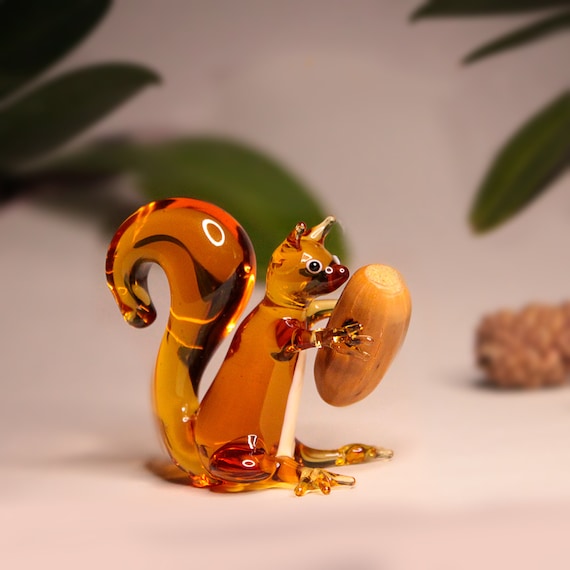This is a detailed color photograph with a square format, capturing an exquisitely detailed blown-glass figurine of a squirrel. The translucent amber-colored squirrel is seated in profile, facing to the right, with its legs tucked underneath and its curved amber tail reflecting a white light from the top right. The squirrel's body, made of see-through resin or plastic, features visible metal joints that allow for articulated hands and feet, each foot having three distinct toes. 

The squirrel's ears are standing up, its nose is a reddish-brown, and it has delicate facial details including distinct eyes and fingers. The squirrel is holding an elliptical, gold-colored acorn that appears to be real, with its front paws grasping the acorn close to its face.

The background is intentionally blurred, featuring large green leafy plants in the top left and right corners, and a brownish piece of rock or similar structure below the leaves in the top right side. The entire composition is set against a cream-colored surface, emphasizing the intricate realism and amber hues of the glass squirrel while maintaining a subtle photographic representationalism realism style.